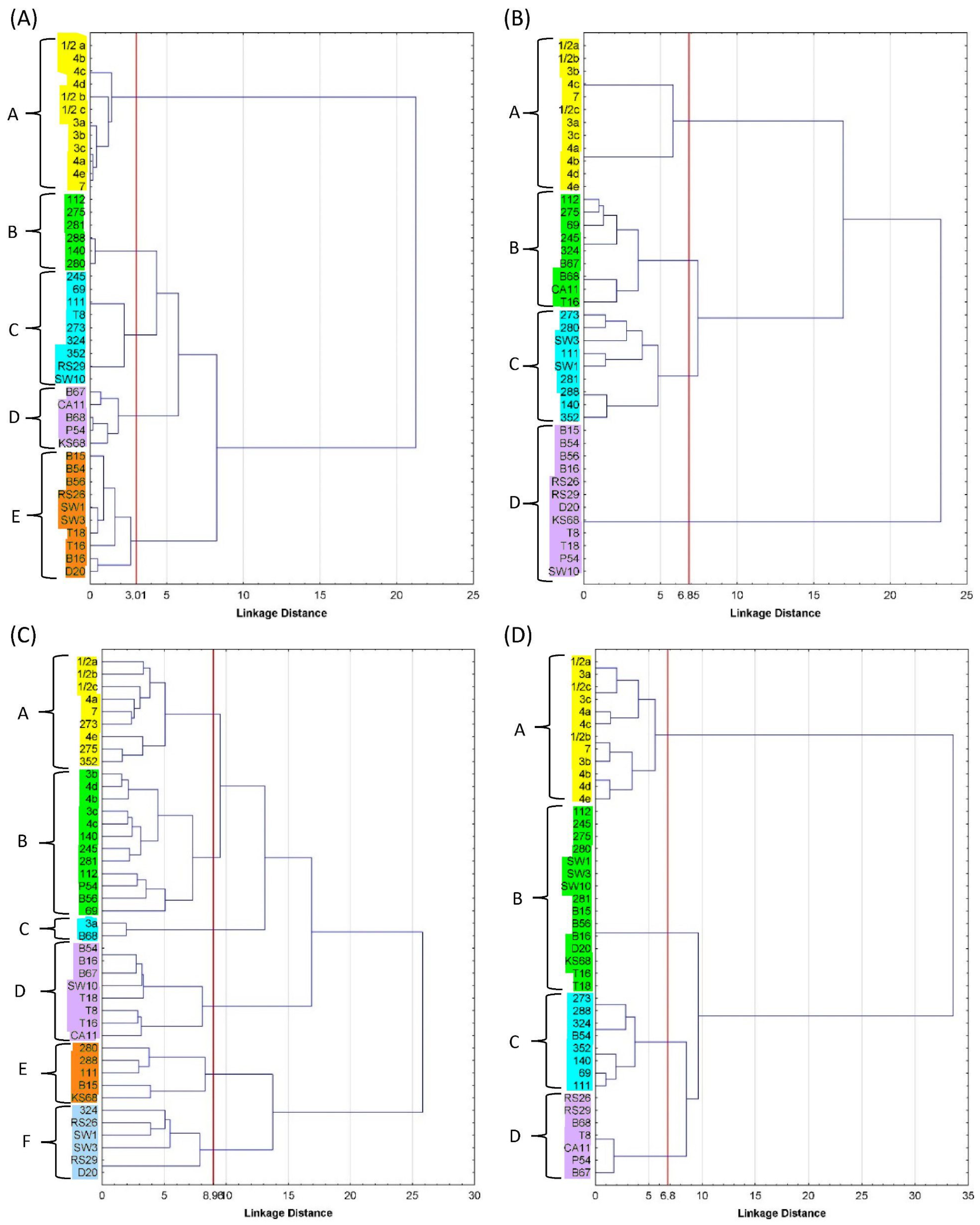The image consists of four distinct graphs organized into a two-by-two grid, with one graph located at the top left, top right, bottom left, and bottom right. Each graph displays a structure reminiscent of tournament brackets, reminiscent of those used in basketball tournaments but applied in a different context. The x-axis of each graph is labeled "Linkage Distance," although the specific units for this measurement are not indicated. The y-axis features a series of labeled segments, denoted by the letters A, B, C, D, and possibly extending to E, each associated with various numerical values.

These graphs illustrate connections between multiple pairs of numbers, linked by vertical lines converging into horizontal lines that subsequently unify with additional numbers, forming complex branching patterns. The structures primarily emphasize clusters and groupings among the A, B, C, and D categories. These intricate linkages suggest relationships or correlations among the numbered entities, although the exact nature or context of these numbers and categories is not provided. Each graph displays a unique pattern of linkages, adding to the complexity and potential insights intended by the visualization.